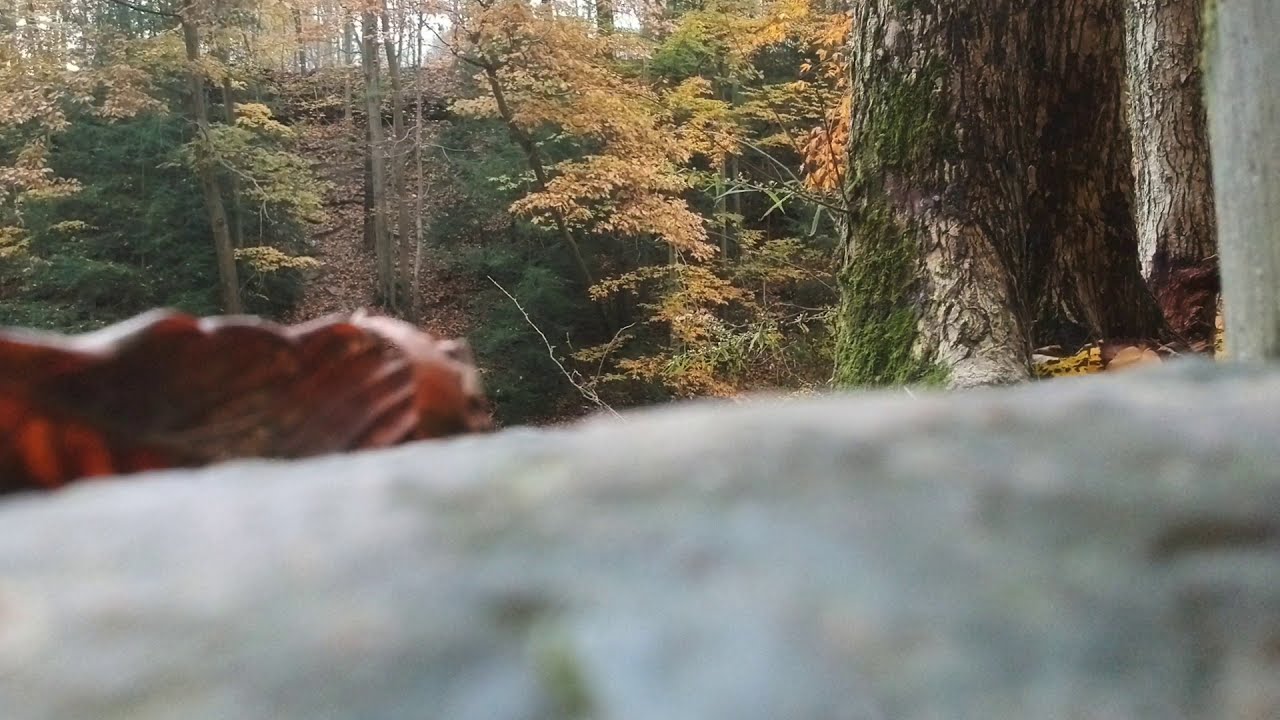The image captures an autumn woodland scene from a low vantage point, as if the photographer is almost lying on the ground. The foreground is dominated by a blurry, light gray surface—possibly a rock or step—which occupies roughly the bottom 20-30% of the photo. Just above this, there is an out-of-focus, reddish-hued leaf towards the center left. The rest of the image is sharply in focus and reveals a richly detailed landscape: 

On the right side, the base of a large tree is adorned with green moss, and two other trees stand nearby. To the left, a ravine or ditch descends the hill, carpeted with orange, yellow, and green leaves. Gray and brown logs with patches of white moss scattered about can also be seen. The ground is strewn with leaves of various colors—primarily orange and yellow—while brown roots snake across the earth. Trees populate the hillside, leading up to a distant tree line that is silhouetted against a sky of blue and white, indicating scattered clouds. The combination of vibrant fall foliage with lingering green life creates a dynamic and picturesque autumnal atmosphere.